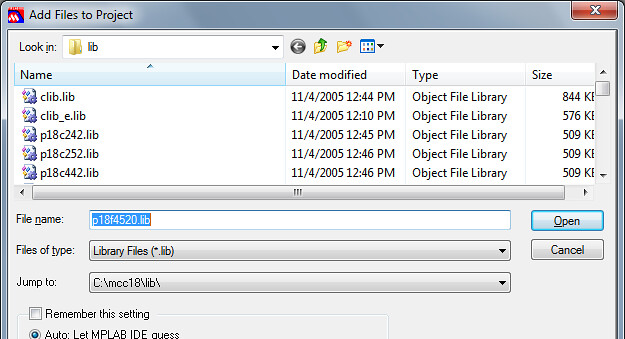This image captures a detailed screenshot of a Windows operating system featuring a pop-up window within a program, likely MPLAB IDE, used for managing project files. The window is predominantly silver-blue and white, embodying typical Windows UI colors. At the top left, there’s a small icon alongside the text "Add files to project," suggesting this window is used for integrating new files into an existing project. This icon is red, blue, and white, but somewhat ambiguous in design. 

The top right of the window features a red 'X' button for closing the dialog. Within the main window, there’s a focus on a folder named "lib," short for library, displaying a list of five object file libraries (.lib). These file names include clip.lib, clip_e.lib, p18c242.lib, p18c252.lib, and p18c442.lib. All files were modified on November 4, 2005—or potentially April 11, 2005, depending on date formatting—during the afternoon hours, with sizes ranging from 500 to 844 kilobytes.

Below the file list, there’s a selection field for "Files of type," set to look for library files (.lib). Additionally, there are options for navigating within the C drive, specifically showing paths like C:\mcc1a\lib. The bottom of the window provides buttons for opening or canceling the operation, a checkbox to remember settings, and another active checkbox labeled "auto: let MPLAB MPLAB IDE guess," reinforcing the likely use of MPLAB IDE software.